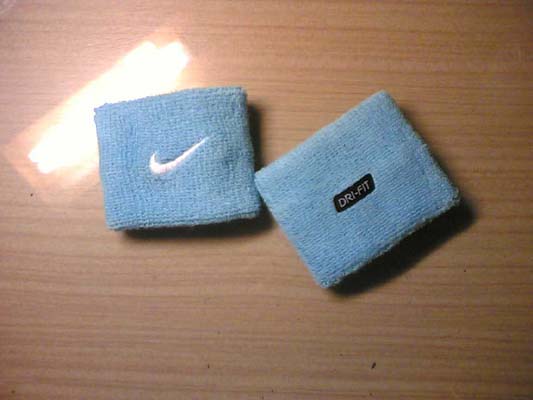The image depicts a light golden brown wooden tabletop with a distinct horizontal grain pattern, illuminated by a bright, rectangular light source, likely an LED, casting reflections and shadows across the surface. Resting centrally on the tabletop are two baby blue, fuzzy-textured sweatbands. The left sweatband features a prominent white Nike swoosh logo, while the right one bears a black rectangular label with "DRI-FIT" written in silver letters. The sweatbands, designed for athletic use such as playing tennis, show some dirt, possibly from prior use, and minor eraser marks can be seen on the tabletop.